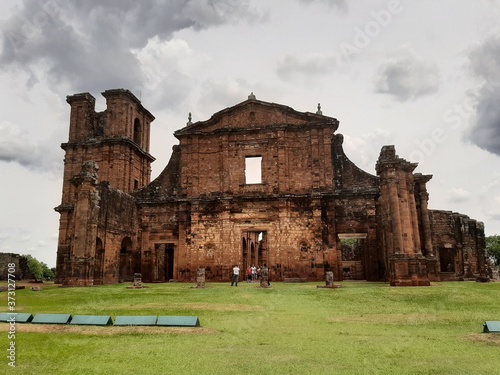The image captures a dilapidated, historical building, possibly an old castle, situated prominently in the middle of the scene. The structure showcases a mix of light and darker shades of brown, illustrating its aged and neglected state. In front of what used to be the main doorway, a group of people is visible, although they appear distant and indistinct. The foreground features a field of short green grass interspersed with dark green, tent-like objects, whose exact nature is unclear. The backdrop is dominated by a gray sky filled with big, puffy clouds, setting a somber tone for the scene. Faint white text reading "Adobe Stock" can be seen, indicating the image's copyright. The color palette includes various shades of gray, white, brown, and green, contributing to the overall atmosphere of historical decay and natural surroundings.